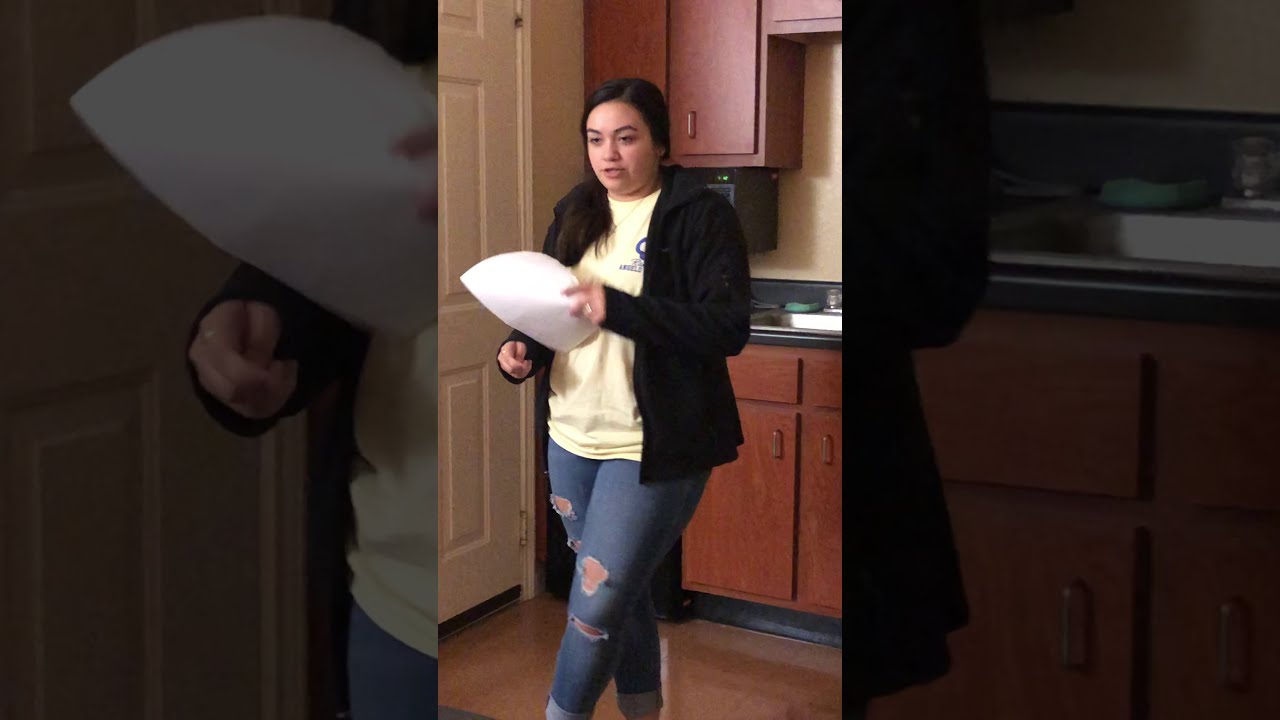The photograph captures a young woman, approximately 17 years old, standing centrally in a kitchen with a white door to her left. She appears to be holding a white piece of paper in her left hand, although it's a bit blurry in that area. Dressed in a black hooded jacket over a white t-shirt and rolled-up ripped blue jeans, she has dark black hair pulled around her right shoulder. She is wearing a ring on her ring finger and her mouth is open as if she is speaking. She stands on brown tiles in front of a sink, which is framed by brown cabinets above and below. The surrounding wall is beige. In the same horizontal rectangular frame, there are close-up images on the left and right sides: the left close-up shows the paper in her hand and part of the door, while the right highlights more of the kitchen sink area and her black jacket. The image exudes a sense of everyday realism, captured in a representational style.